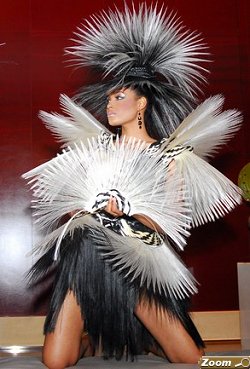This full-color photograph captures a striking scene of a model, possibly of light African or Middle Eastern descent, kneeling on a gray rug against a maroon backdrop, likely during a fashion show. She is adorned in a dramatic and elaborate feathered outfit with a cohesive color scheme of black, white, and gray. The ensemble includes a top with white, upward-pointing spiky feather epaulets, a black feather skirt, and a grand, long feathered headdress. Complementing her outfit, she holds a fan crafted from matching feathers. The model's head is turned to the left, showcasing her white eyeshadow and elegant earrings, enhancing her overall majestic and ethereal appearance.